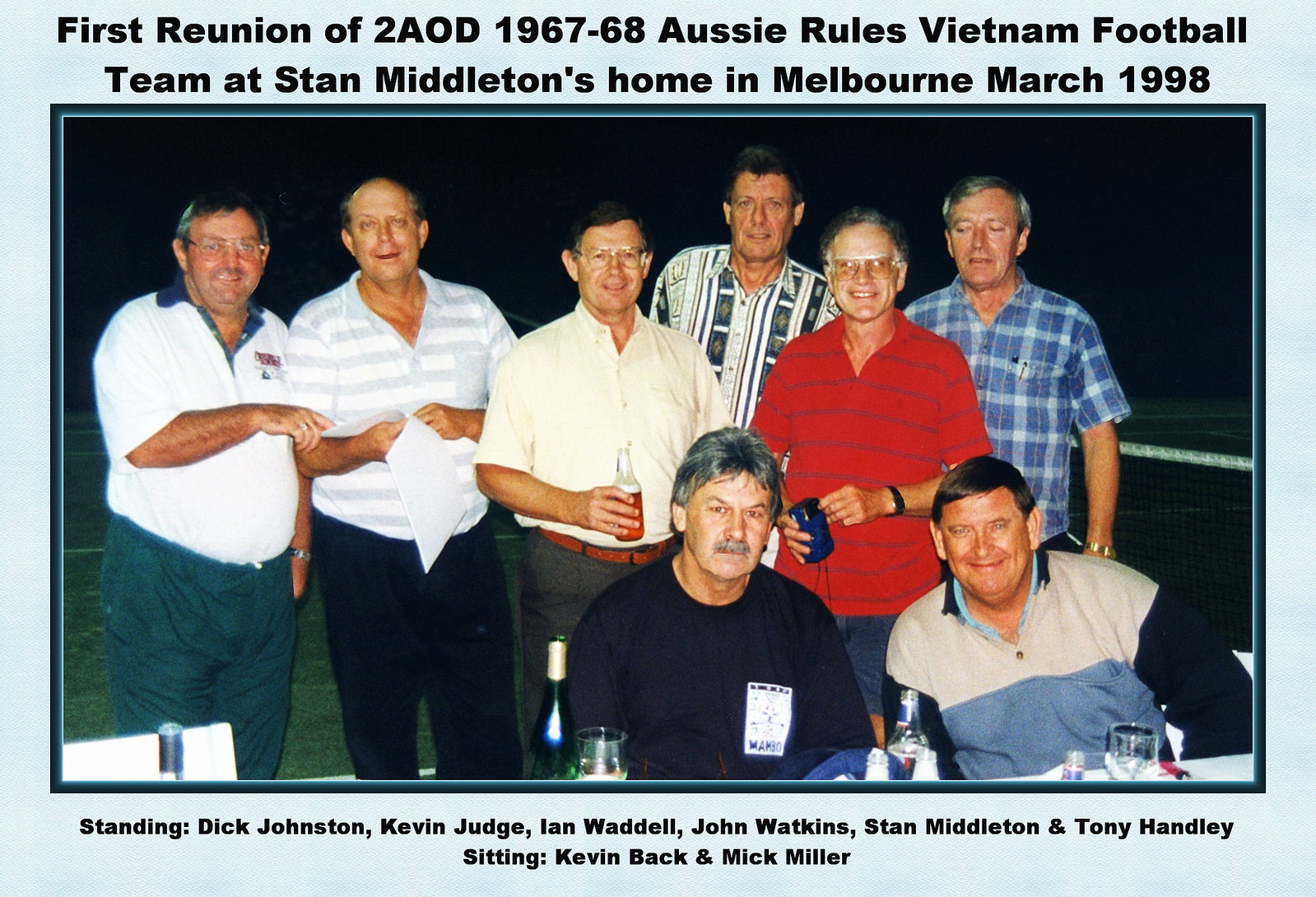This photograph, bordered in light blue, captures a lively gathering of eight older men, presumably sharing a warm reunion. The caption across the top reads: "First Reunion of 2AOD 1967-68, Aussie Rules Vietnam Football Team at Stan Middleton's Home in Melbourne, March 1998," while the bottom border lists their names: "Standing, Dick Johnston, Kevin Judge, Ian Waddle, John Watkins, Stan Middleton, and Tony Hadley. Sitting, Kevin Beck, and Mick Miller."

Starting from the left, a man in a white shirt and light blue pants points towards the right. Beside him, another man clad in a white shirt with gray stripes and black pants looks forward. The third man, wearing a yellow shirt and glasses, has black hair and gray pants with a belt. Behind them all stands another man with black hair, dressed in a vertical-striped button-up shirt. On the right, a man in a red T-shirt, glasses, black watch, and holding a blue cup, is visible. In the back, an elderly man dons a plaid blue shirt and appears to have his eyes closed. In the front row, two men are seated: one in a dark blue long-sleeve sweatshirt, with gray and black hair and a mustache, and the other sporting black hair and smiling, wearing a shirt that is gray on top with blue sleeves and the words "First Reunion of AOD 1967-68" written across it.

The men seem relaxed and cheerful, gathered outdoors, possibly enjoying drinks together as suggested by the presence of beers, empty glasses, and a champagne bottle on the table before them. The photograph, illuminated perhaps by a camera flash, exudes an atmosphere of nostalgia and camaraderie among the well-dressed, mostly gray-haired participants of this memorable event.